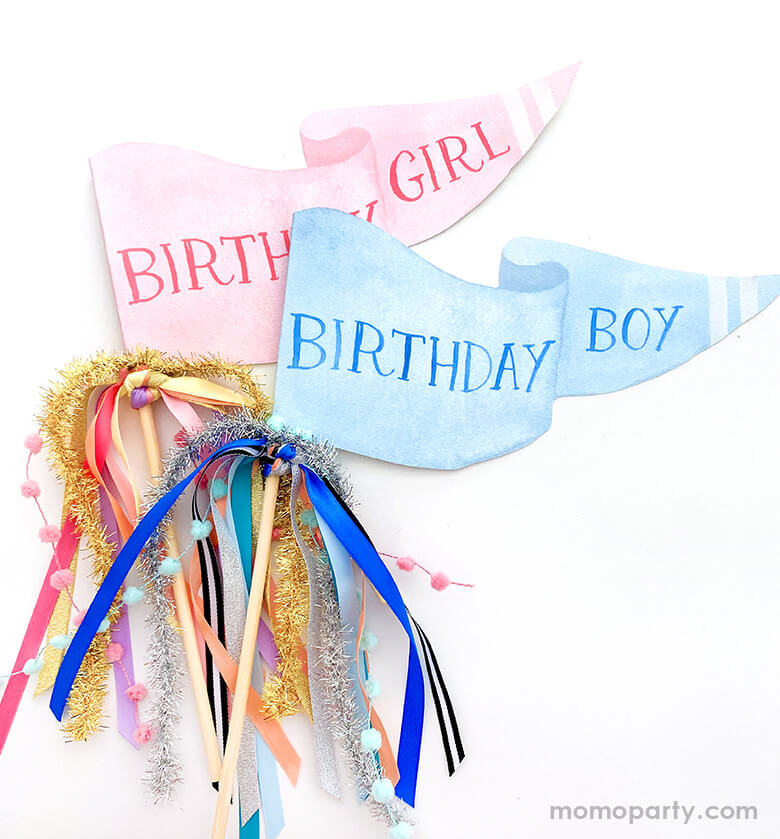The image, courtesy of momoparty.com, features two small, triangular flags against a white background. The first flag is blue with the words "Birthday Boy" written in a solid blue hue, reminiscent of a watercolor effect. The second flag is pink with "Birthday Girl" inscribed in a reddish-pink on the also watercolor-like light pink background. Both flags are attached to wooden sticks, resembling the look of wooden skewers. Adorning the sticks are various multicolored ribbons and tinsel-like embellishments. The blue flag boasts blue and white pompoms along with blue, white, and black streamers, while the pink flag is decorated with gold, pink, yellow, and purple ribbons, coupled with pink and white pompoms. Additionally, the sticks of the flags are twined with gold and silver tassels, enhancing their festive appearance. The momoparty.com website address is subtly placed in the bottom right corner of the image, colored in gray.